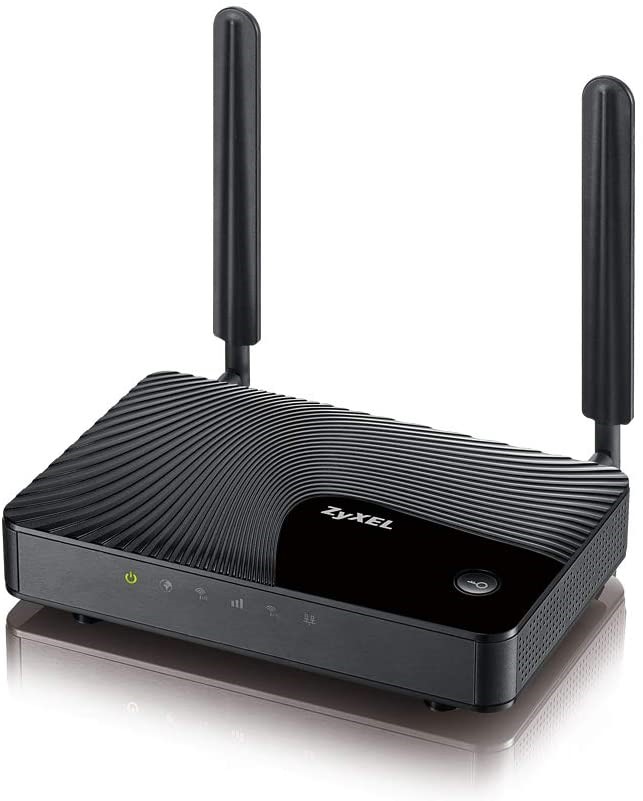The image is a detailed stock photograph or advertisement featuring a router, specifically a Zyxel model, placed against a white background. The router is a small, rectangular, gray and black device with a unique wavy design that wraps around its sides and front. It is positioned at a 30 to 45-degree angle to the left from the viewer's perspective, with the bottom right-hand corner closer to the camera. The top of the white stand it is placed on is barely visible. 

The router features two black plastic antennas that resemble paddle handles, rising from the back corners and extending upwards, estimated to be about 8 to 10 inches long. On the top, within a black oval-shaped area, the brand name "Zyxel" is prominently displayed. The area also houses a green, lit power button on the right. Along the front of the device, several indicator lights can be seen, including symbols for power, a globe, Wi-Fi connectivity, and three vertical bars indicating signal strength. Additionally, there are a couple of unidentified symbols at the far right of the display. The overall design includes many cooling fins and intricate patterns on the top, providing both functionality and a modern aesthetic.